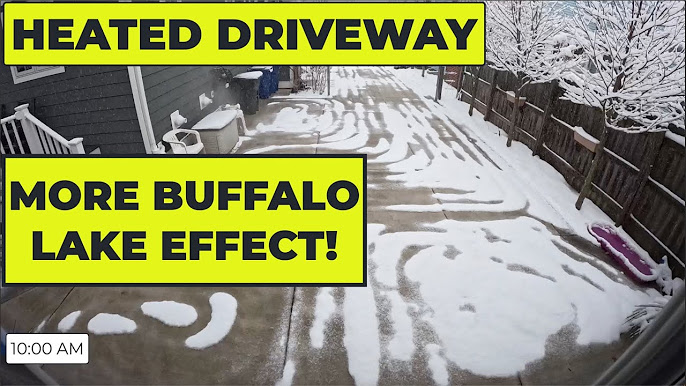The image is a YouTube thumbnail showcasing a heated driveway, designed to demonstrate the effectiveness of the heating system in melting snow. The thumbnail prominently features text in black font against high-visibility yellow backgrounds, with "Heated Driveway" displayed at the top and "More Buffalo Lake Effect" right below it. Additionally, "10 a.m." is noted in the bottom left corner, suggesting the time of observation.

In the scene, the driveway is partially covered with snow, visibly melting away due to the heating system. Surrounding this area, a brown privacy fence lines the right side of the image, adorned with snow-covered trees. On the left side, a dark-sided house with white trims and steps is visible, featuring a white window. The driveway contains some salt residue from melted snow and includes various items such as a purple cart or board in the lower right corner, trash cans near the house wall, and possibly some outdoor patio furniture. The composition captures a real-world application of the heated driveway, emphasizing its practicality during snowy conditions.